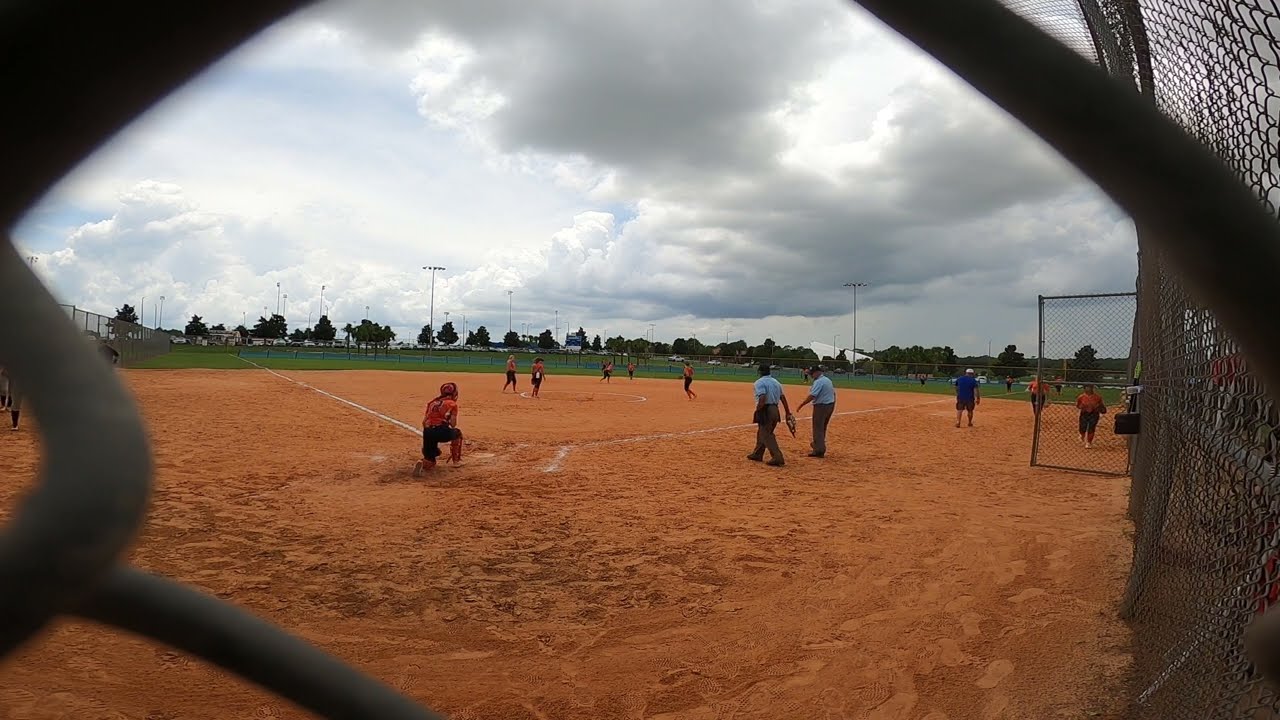This photograph captures a vivid and dynamic scene of a baseball game from the unique vantage point of behind a metal fence, with the diamond-patterned grates partially framing the image. Taken from behind the catcher, who is kneeling at home plate wearing a red jersey, the image shows the well-trodden, orange-brown soil of the playing field. Several players in red and black uniforms are scattered across the field, with one positioned on the mound and another approaching it. There are also two umpires present, distinguished by their light blue shirts, seemingly in discussion. The outfield transitions from the earthy infield to lush green grass, stretching towards the horizon where trees are visible. Above, the sky is a mix of blue and cloud cover, adding to the sense of a slightly overcast day. Beyond the field, some people can be seen walking around, contributing to the active atmosphere of the park.